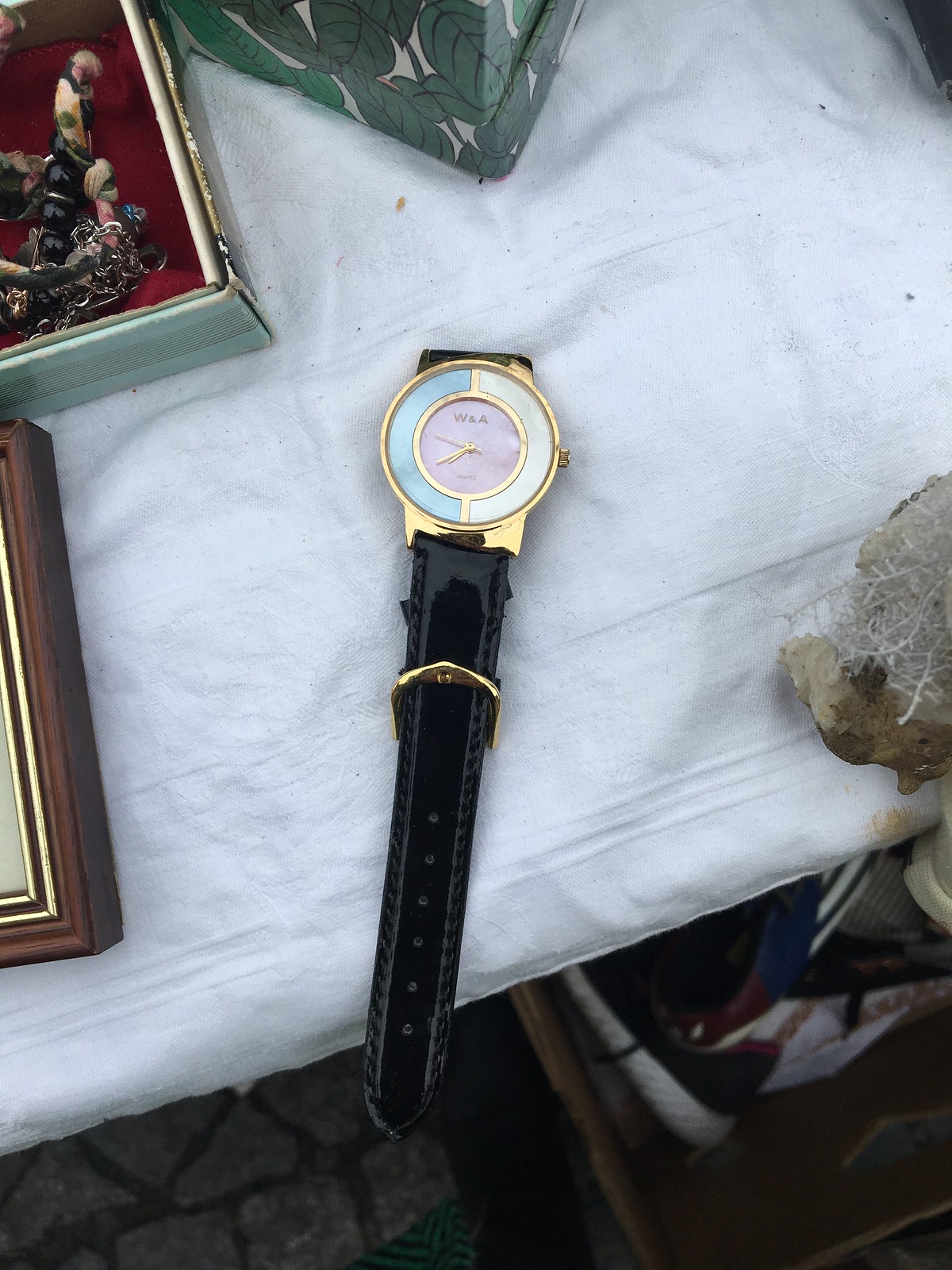This is a close-up, vertically-oriented photograph of a meticulously detailed women's watch, captivatingly placed on a white tablecloth that bears a few dirt and black spots, possibly at a yard sale. The watch has a black patent leather strap featuring many small circles and a gold clasp. Its circular face encased in a gold bezel, showcases intricate details: a light blue 'C' shape facing a cream-colored 'C', separated by a slender vertical gold piece, with a central inner circle in pink, all accentuated by gold hands displaying the time around 7:41 and 50 seconds. Surrounding the watch are various items indicating a yard sale setting, including a dark chocolate brown wooden box outlined in lighter brown, a gray rock with white web-like material on top, a box with a green leaf-patterned border with a beige background, and a light blue box with a maroon-belted interior housing assorted jewelry. Also present is a brown picture frame with gold trim and a cream-colored picture on the left edge, partially out of frame, and other items including a red velvet box containing bracelets and earrings, all laid out on the table amidst a backdrop of diverse objects and colors.